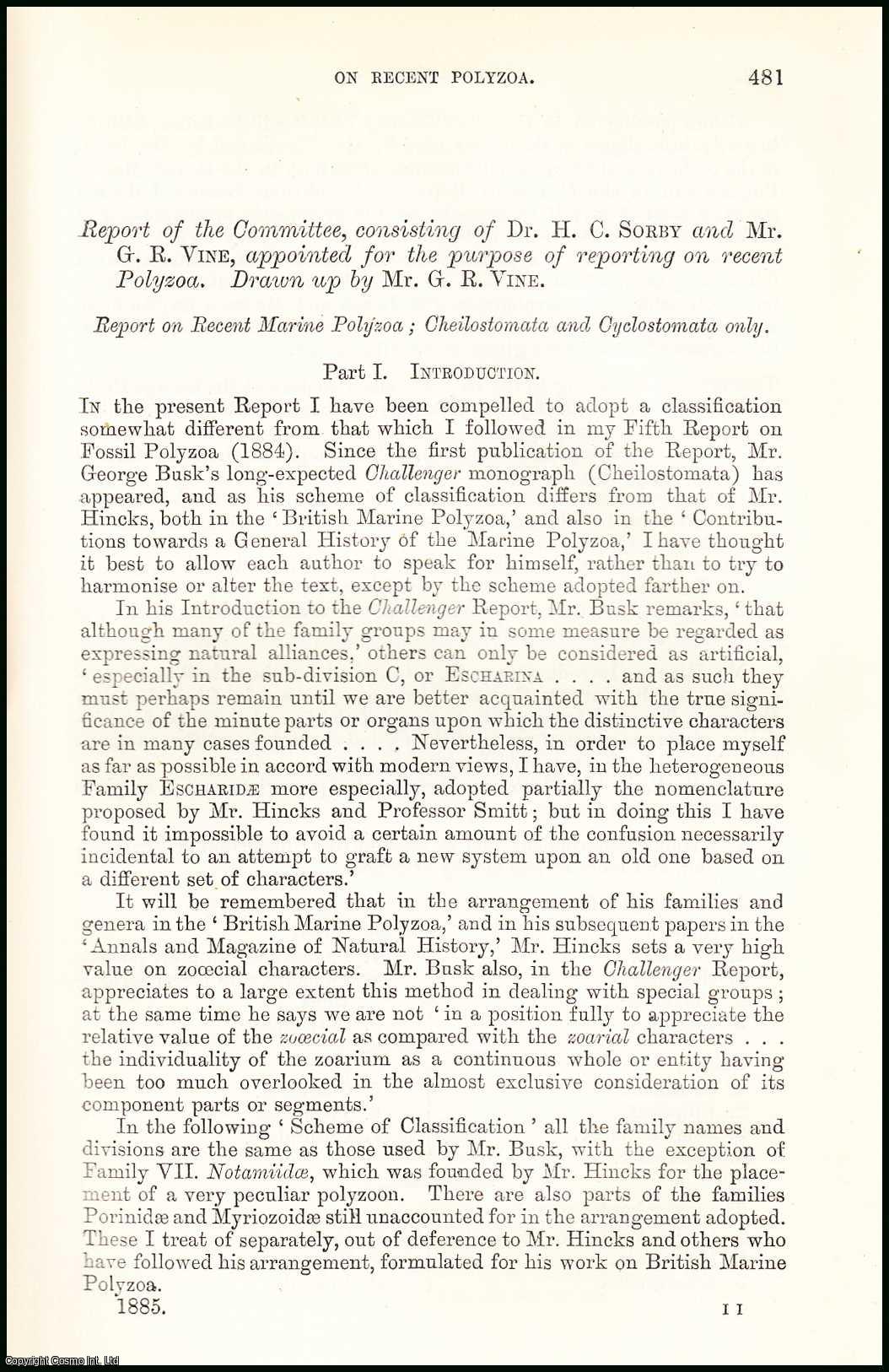The image is a photograph of an old document, resembling historical documents such as the Declaration of Independence. The document appears to be a typewritten or scanned page, possibly from the 1800s, judging by its style and the challenges posed by the faded font. The title reads "Report of the Committee," specifically noting the involvement of Dr. H.C. Sorby and Mr. G.R. Vine. They were appointed to report on "Recent Polyzoa" and the document states, "Drawn up by Mr. G.R. Vine." It focuses on recent marine polyzoa, particularly Chilostomata and Cyclostomata. The page, numbered 481 at the top right, appears as an introduction, citing that it builds upon a previous report from 1884, with evidence suggesting the current date is 1885. The legibility is compromised, making it difficult to discern all the sentences, but it distinctly marks this as part one of their findings.